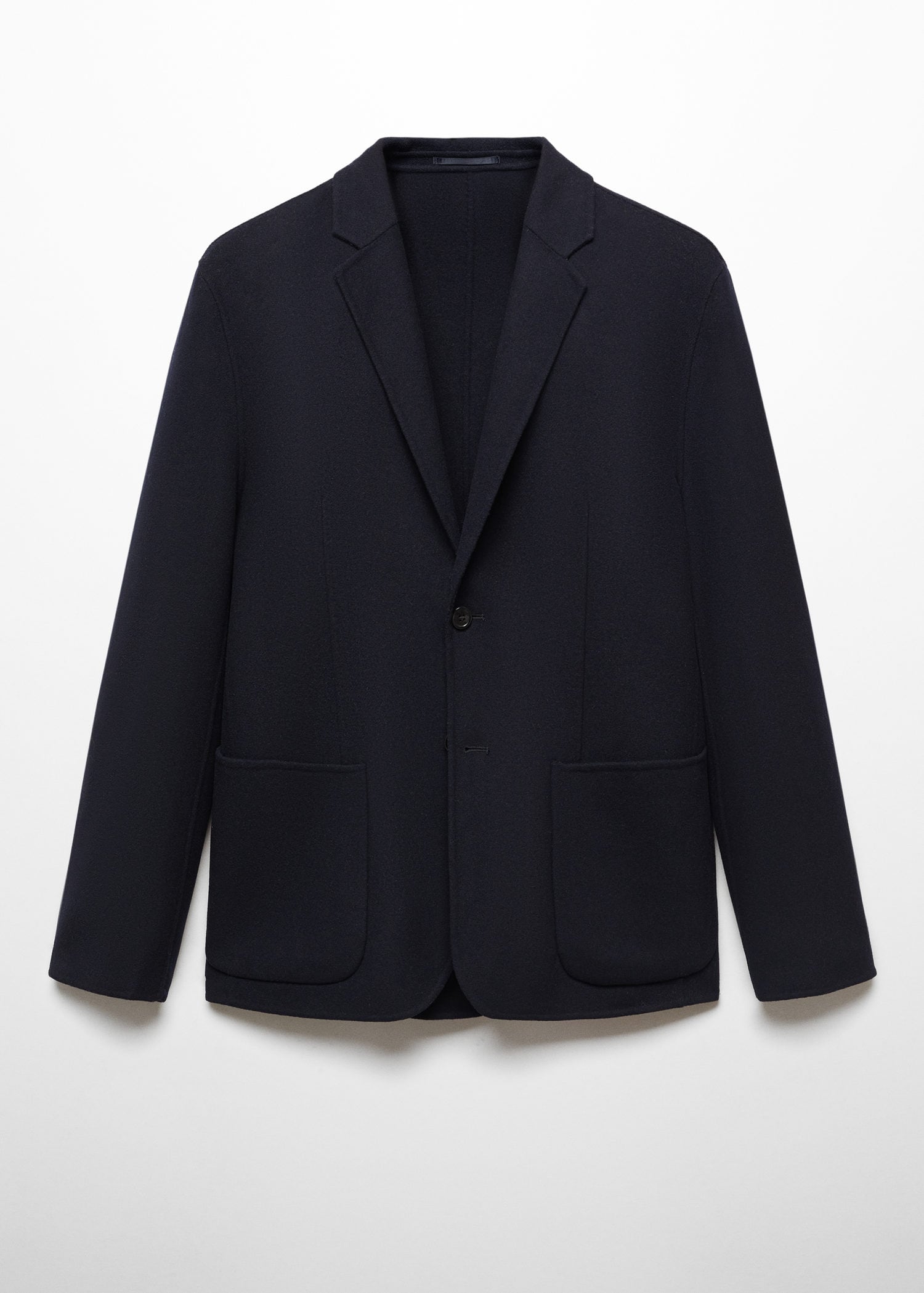The image features a sophisticated, all-black wool blazer, centered against a plain white background. The jacket, which could be for either men or women, exudes a minimalist and elegant design. It sports a folded collar and a single button positioned halfway up the torso. Two deep pockets are sewn symmetrically on either side of the front. The jacket's interior matches the same rich black color and material as the exterior, emphasizing its cohesive and sleek look. This versatile and refined blazer can effortlessly complement any outfit, making it suitable for both casual and formal occasions.